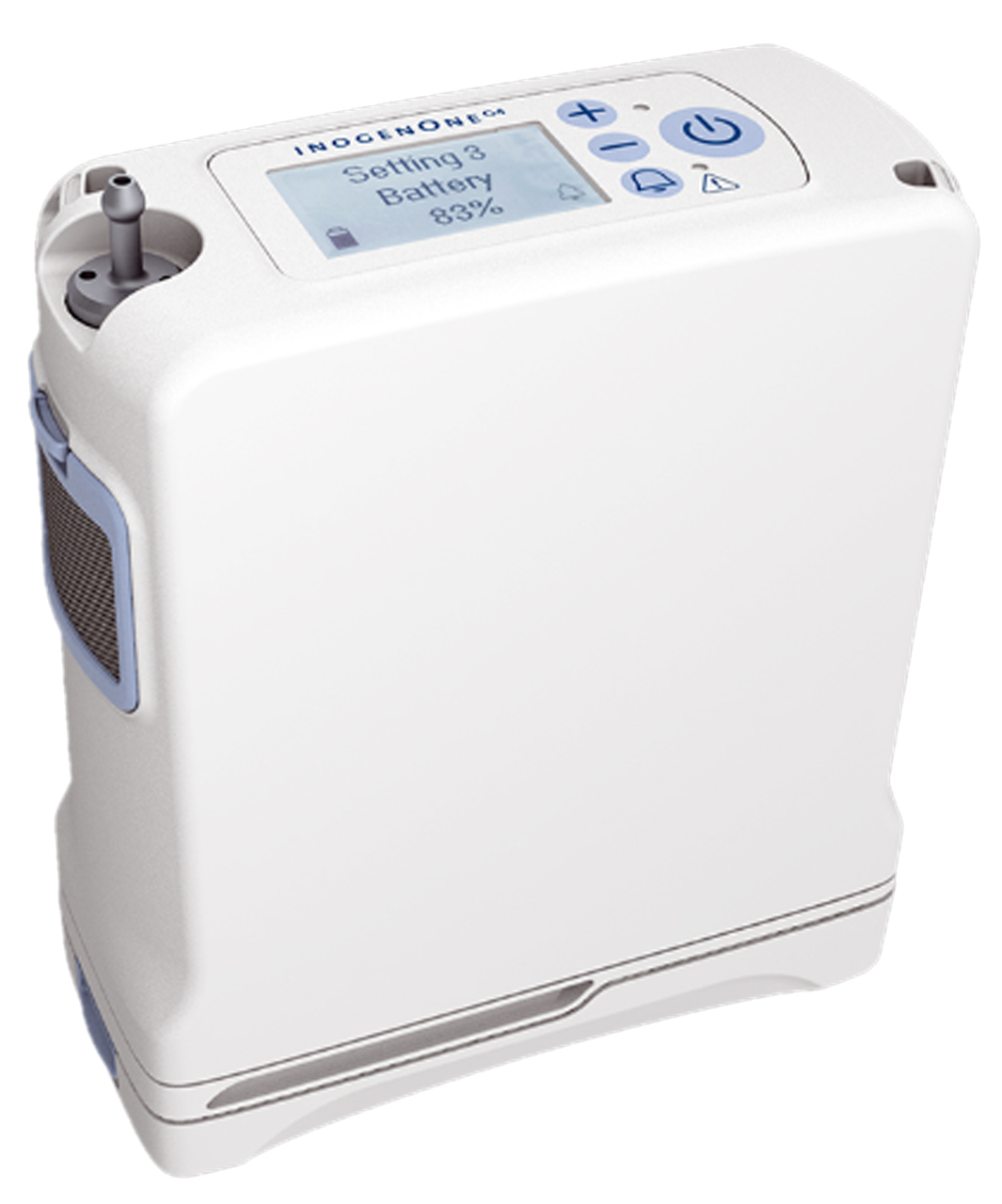The image showcases a rectangular, white device resembling a compact computer tower, identified as an Inogen One G4. A gray handle is situated at the top left, and next to it, an upper-left side panel is noted to be light blue with a small notch, suggesting it is removable. A display screen at the top center reads "setting 3, battery 83%." Above this screen, the brand name "Inogen One" is prominently displayed. To the right of the display are blue control buttons featuring a plus sign, a minus sign, a bell icon, and a large power button marked with a circle and line design. Additionally, a warning triangle with an exclamation point is present beneath the power button. The front of the device includes a filter and a nozzle, hinting at its function as an air purifier or oxygen concentrator. The device stands on a metallic part, serving as its base. The unique design combines practical features with a modern aesthetic.